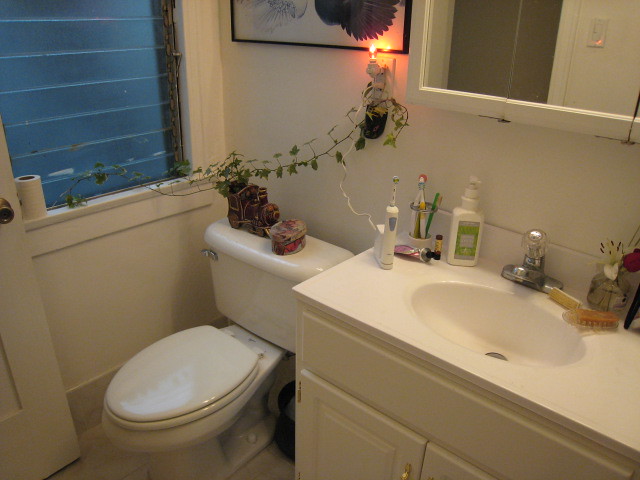The image showcases a well-kept bathroom with an organized and tidy setup. To the right side of the image, we see a sleek white sink mounted on a white counter. Below the sink, there are two spacious white cabinets providing storage space. On the left side of the sink, an electric toothbrush stands next to a cup brimming with regular toothbrushes. Just below these items lies a tube, while a bottle of hand soap is positioned on the right side of the sink. Adjacent to the soap, a decorative vase holding a fresh bouquet of flowers adds a touch of nature, accompanied by a cleaning sponge and a brush.

Above the sink, a mirror with a built-in cabinet graces the wall, offering both reflection and additional storage. Moving towards the left end of the counter, a standard white toilet with a wide handle is placed neatly against the wall. A charming small vine plant drapes overhead, its left end resting on the windowsill to the left of the toilet, while its right end hangs from an electrical outlet located just above the toilet. The outlet also supports a brightly lit nightlight, providing a gentle glow to the bathroom space.